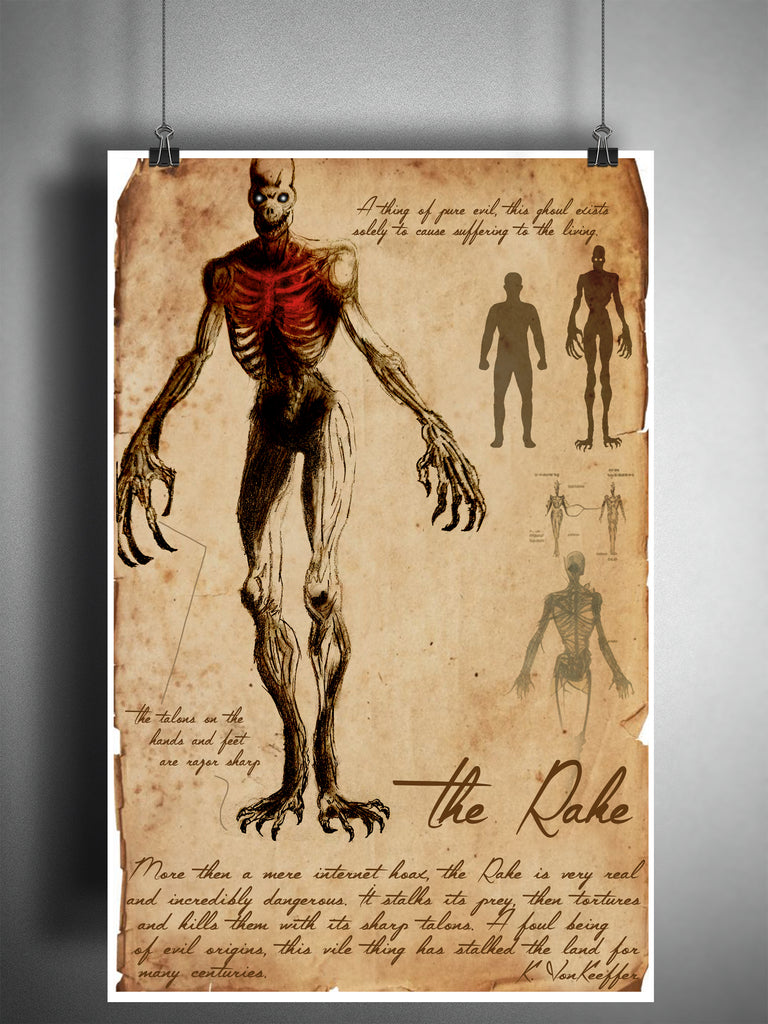This image presents a detailed drawing of a creature known as the Rake, depicted on a vintage, brown-aged piece of paper with a white border. The painting is suspended in mid-air, held up by two wires that have black clamps at the corners. The backdrop is a gray wall, slightly shadowed by the paper.

The Rake is portrayed as a grotesque, skeletal creature with a dog-like skull, its mouth slightly ajar revealing black eyes with white pupils. Its gaunt frame prominently displays an exposed ribcage with red bones, further emphasizing its monstrous nature. The arms extend downward and outward with long, black fingers that are slightly bent. The legs appear muscular yet skeletal, extending to black and white clawed feet shaped like talons, each bearing almost five fingers. 

In the lower right corner of the image, the term "The Rake" is written in bold black lettering, accompanied by a paragraph describing its sinister nature. Above to the right, shadows of a human and the Rake are cast, highlighting the creature's towering stature, at least two feet taller than the human figure. The detailed depiction and accompanying text suggest an eerie, historical lore surrounding the Rake, emphasizing its long-standing presence and perilous reputation as a malevolent stalker.